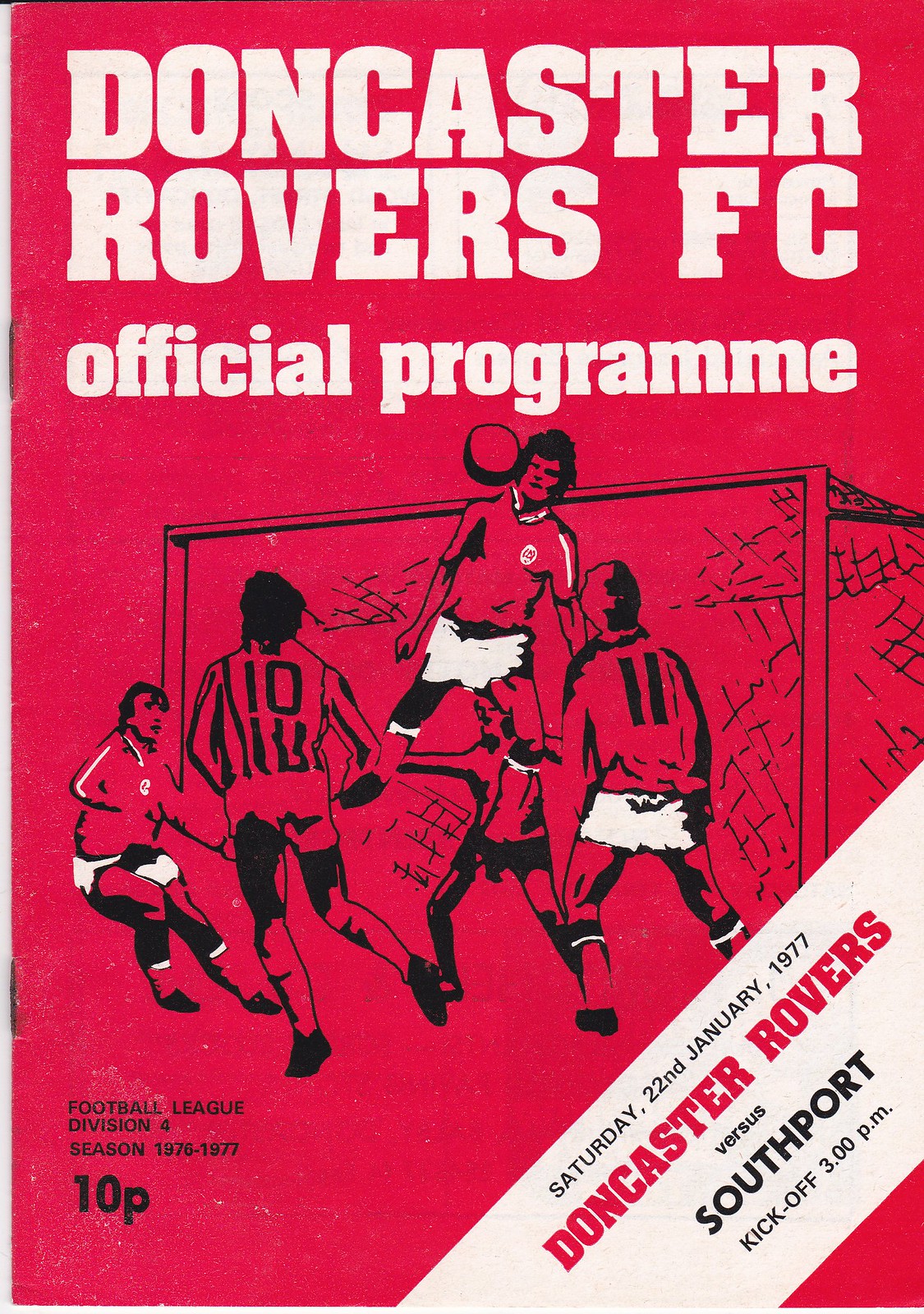The cover of the official program for the Doncaster Rovers FC Football League match from January 22, 1977, features a vivid red background with detailed black line art illustration. Central to the image is a dynamic scene in front of the goal net, capturing five players mid-game, including the goalie who is airborne as he attempts to head the ball. Among the players, one is wearing a jersey with the number 10, and another with number 11. The top of the cover displays 'DONCASTER ROVERS FC' in bold white capital letters, followed by 'official program' in lowercase. A white diagonal stripe on the lower right side provides game details in black and red text, noting 'Saturday 22nd January 1977, Doncaster Rovers versus Southport, kickoff 3 p.m.' In the bottom left corner, small black text reads 'Football League Division 4, season 1976-1977, 10p.' Additionally, two metal staples are visible along the program's left edge.